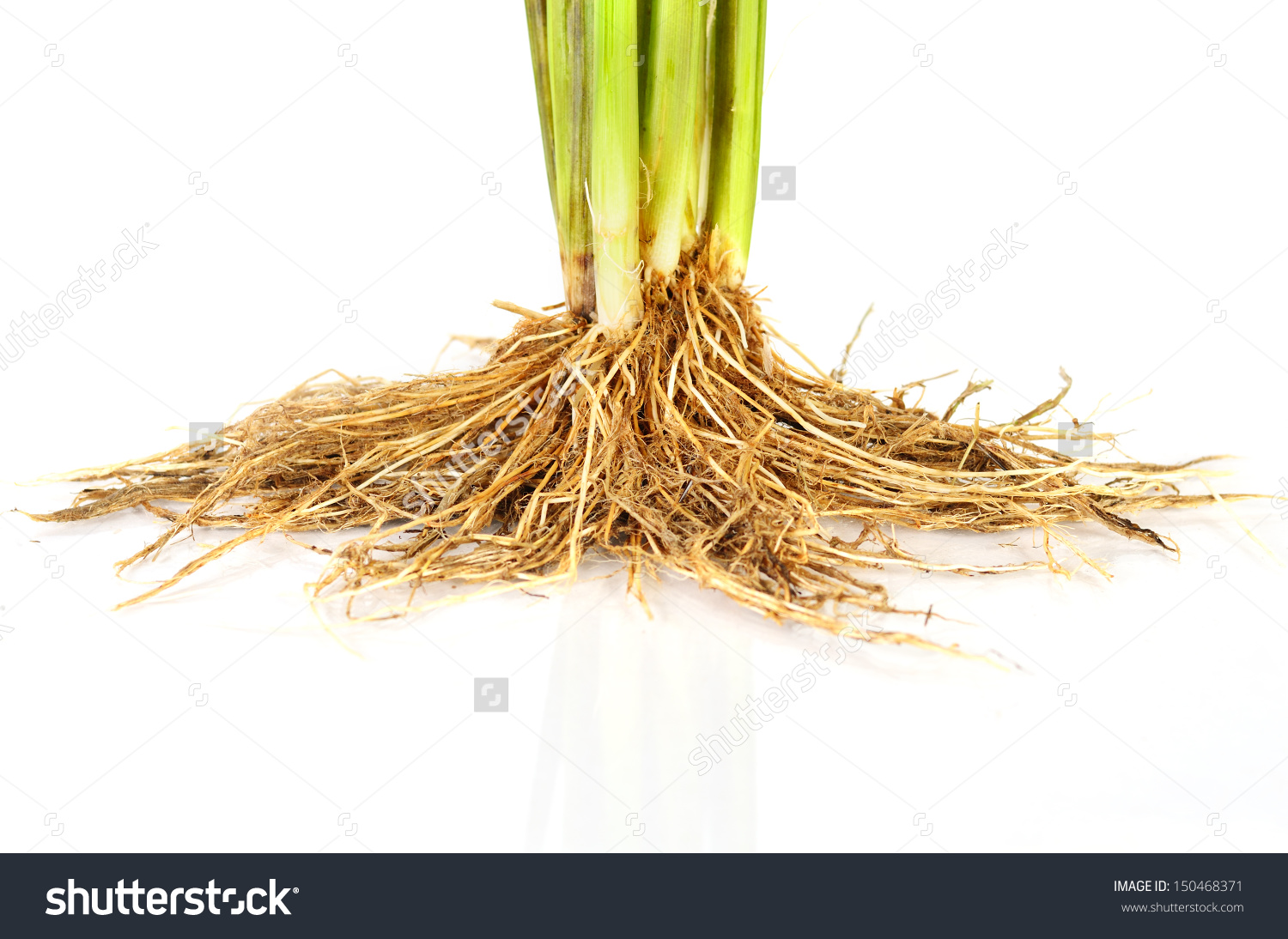The image showcases a close-up view of what appears to be green onions with slightly brown and shriveled tops. The bright green stalks, turning white near the base, are standing upright, while a dense network of thousands of tan, beige, and brown fibrous roots spreads out beneath them. Some roots extend horizontally to the left and right, with others forming a V-shape in the front, creating a sprawling display. Tiny bits of dirt cling to the roots, suggesting they were recently pulled from the ground. The background is white, and the image is watermarked multiple times with the text "Shutterstock." At the bottom, a black band bears white text that includes the Shutterstock logo, an image ID number, and a website address.